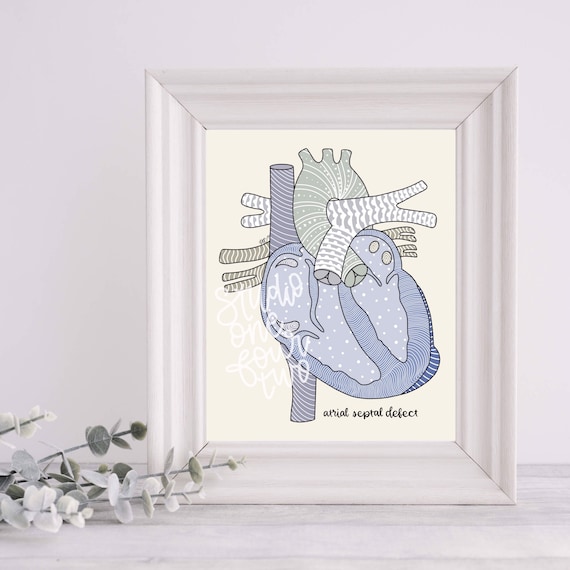The image depicts a framed piece of artwork featuring a stylized, cross-sectional illustration of a human heart. The heart is primarily colored in light blue, green, and white, against a light yellow background, giving it a somewhat muted, toned-down appearance. This heart illustration, which appears almost cartoonish, is centered within a white wooden frame. In the lower right-hand corner of the artwork, there is some black text that reads "atrial septal defect," and white text above that says "Studio 142." The framed artwork is positioned against a white background, resting on what seems to be a white wooden table or shelf. To the left of the frame, there are partially visible accents of fake white-leaved plants, which add a decorative element to the scene.